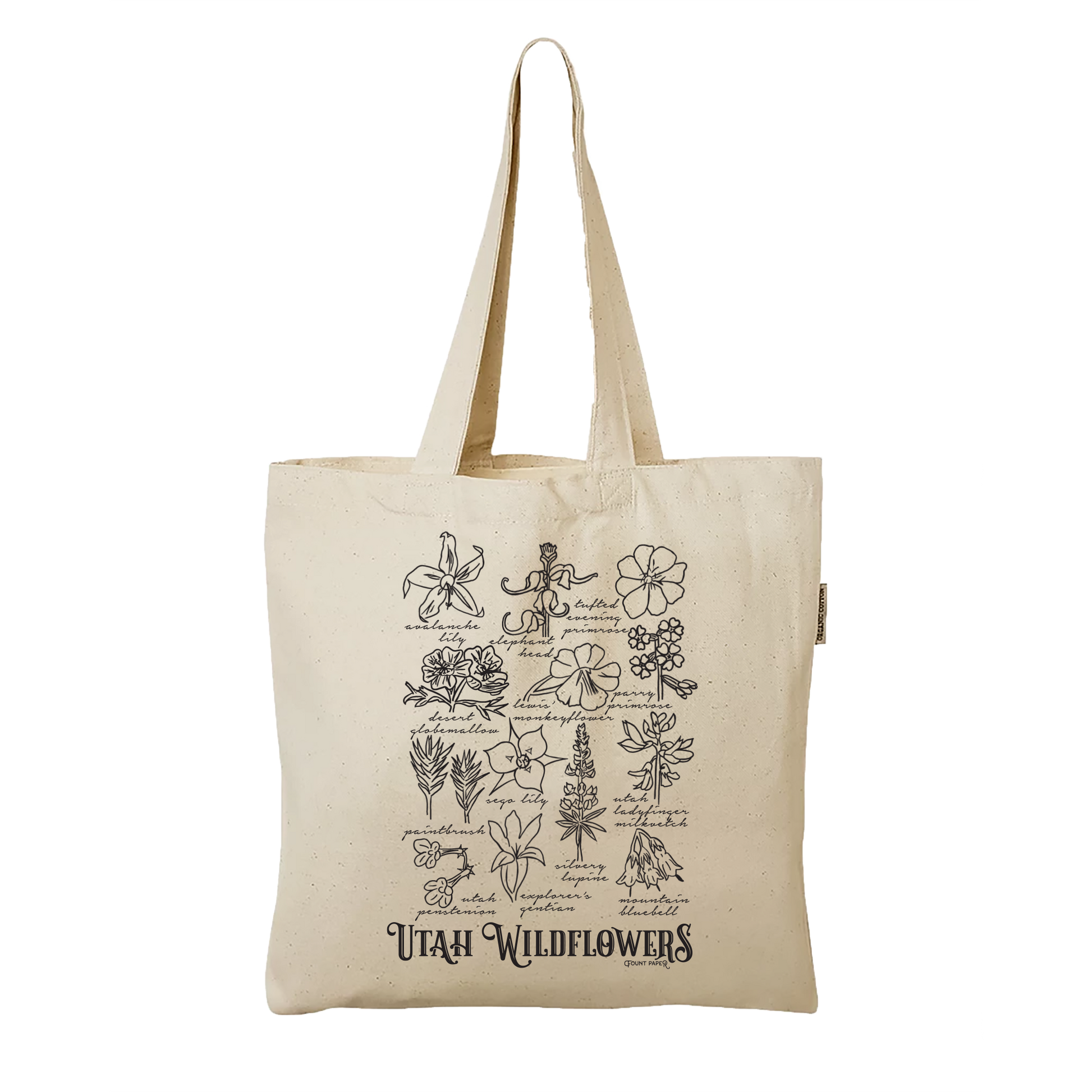The image depicts a cream-colored canvas tote bag against a white background. The tote bag features two looping handles and a nearly square shape. On the bag, there are black hand-drawn sketches of various Utah wildflowers including examples like Avalanche Lily, Paintbrush, Explorer's Gentian, Mountain Bluebell, and Elephant Head. Each flower is accompanied by its name written in cursive beneath the sketch. At the bottom of these illustrations, in all capital letters, the text reads "UTAH WILDFLOWERS." The overall design is simplistic with black and white graphics on a light tan fabric, highlighting around 12 to 13 different species of Utah's wildflowers.